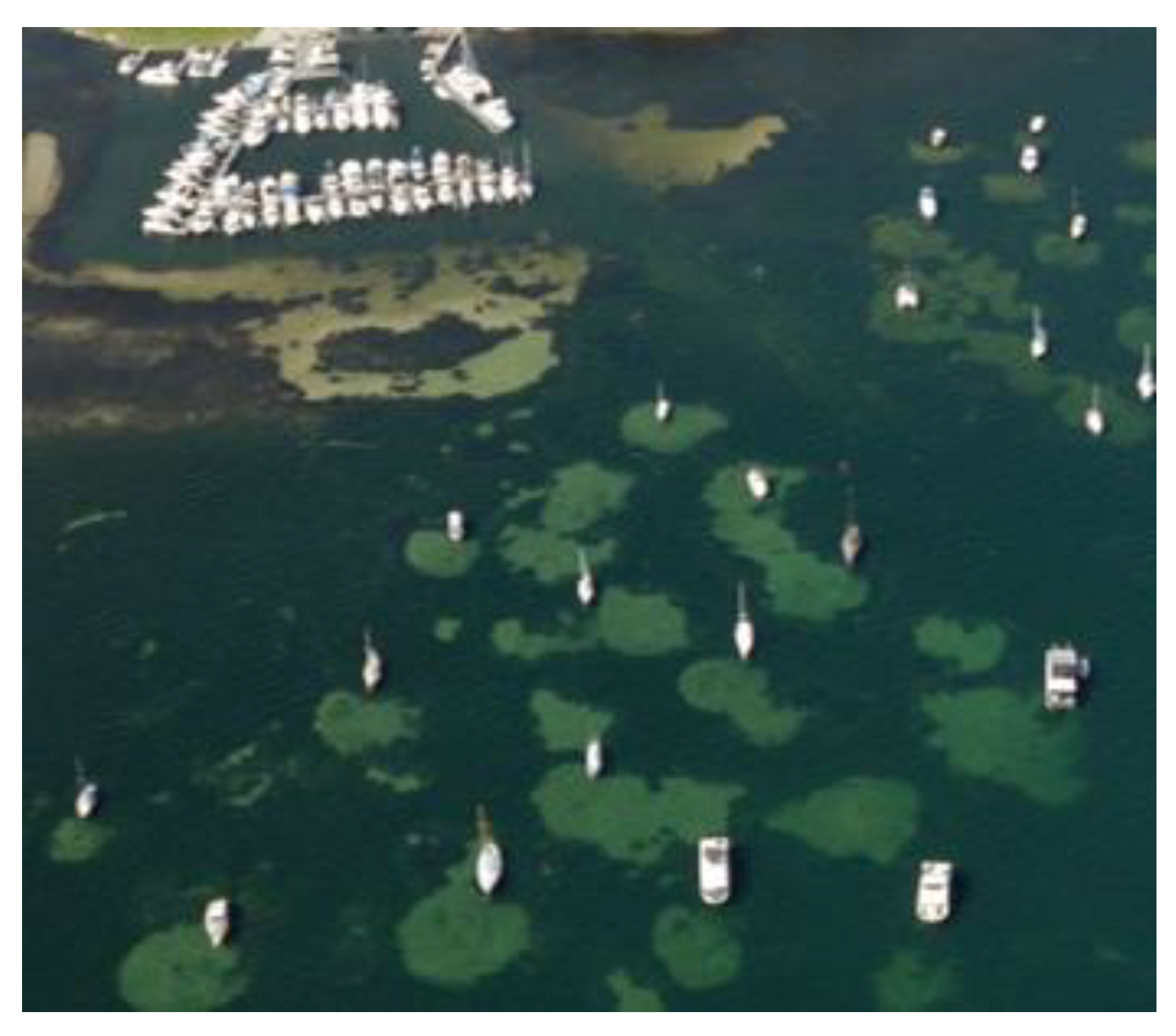A slightly blurred daytime image depicts a coastal marina with numerous white boats of varying sizes and shapes, some rectangular and others more triangular. The boats, spaced evenly apart, appear to be heading toward the bottom of the image, navigating through greenish-blue waters that reveal submerged patches of land. In the top left corner, a ship dockyard or bay area is visible, with multiple boats docked. The largest boat, approximately three times the length of the average boat, is seen on the right side of the marina, identifiable by its distinctive length and the presence of blue and cyan canopies on several boats.